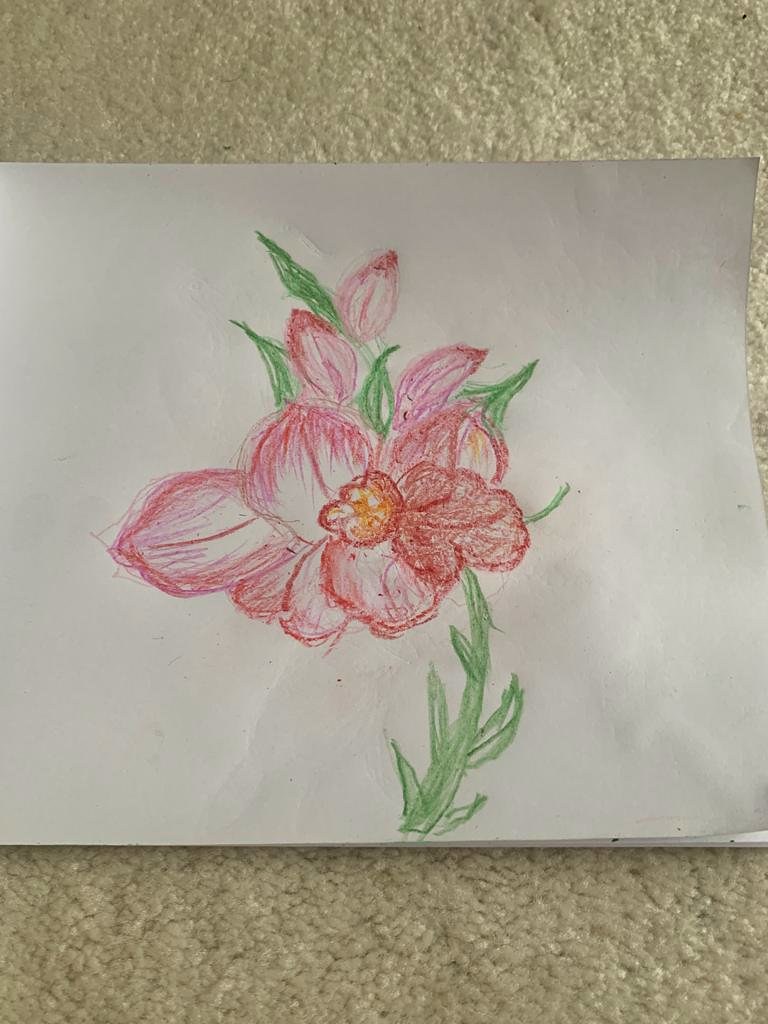This photograph captures a colored pencil drawing of a red flower with a green stem and leaves, created on a worn piece of white paper. The flower, featuring about a dozen red petals with hints of orange or yellow at the center, is simply yet attractively drawn. The light green stem is adorned with pinkish-edged, white-centered leaves, arranged on either side as it ascends to the flower. The naïve, somewhat crude sketch appears to have been done by an amateur, possibly a child. The well-worn paper, bearing multiple creases and imprints from previous writings, rests on an off-white, beige-like carpet, adding to the casual, authentic feel of the artwork.